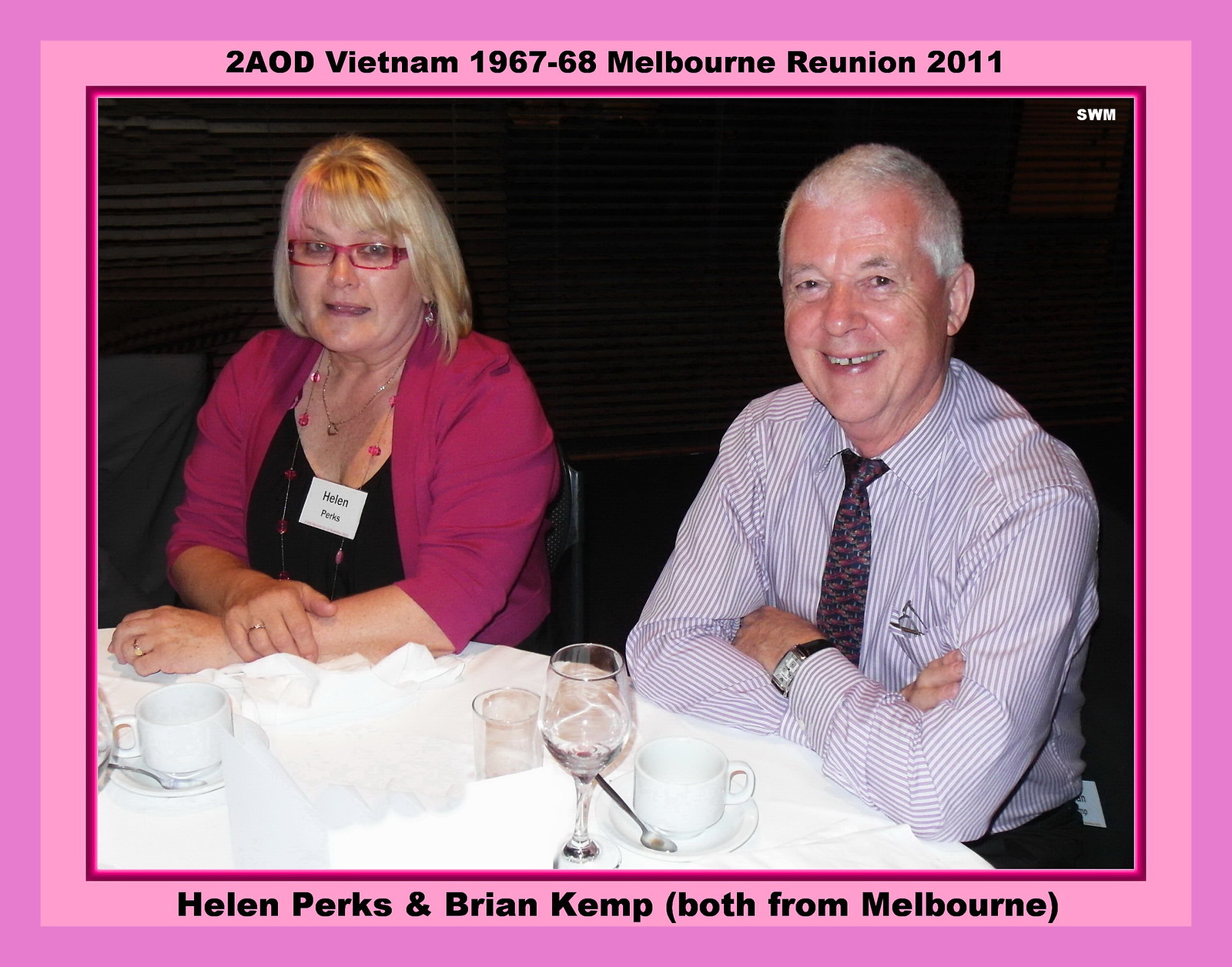This photograph captures a moment between two individuals, a man and a woman, seated at a round table covered with a white tablecloth in what appears to be a restaurant. Both are looking directly at the camera. The man, seated on the right, is a white man with short white hair, wearing a white shirt with black vertical stripes and a black and pink tie. His arms are resting on the table with his elbows. In front of him, a white coffee cup and saucer, as well as a wine glass filled with water, are visible. The woman, seated on the left, has shoulder-length straight blonde hair and is wearing pink rectangular glasses. She is clad in a black blouse underneath a pink jacket and has a white name tag that reads "Helen Perks." Her arms are also resting on the table, and in front of her is a white coffee cup and saucer, both with silver spoons.

Surrounding the photograph is a triple-border frame. The innermost border is thin and dark pink. Above the photograph, the thicker, light pink middle border features the text: "2AOD, Vietnam, 1967-68, Melbourne Reunion, 2011." The bottom of this border reads: "Helen Perks and Brian Kemp, both from Melbourne." The outermost border is a dark pink shade. The background behind the two subjects is notably dark, providing a contrast that ensures the subjects are the focal point of the image.